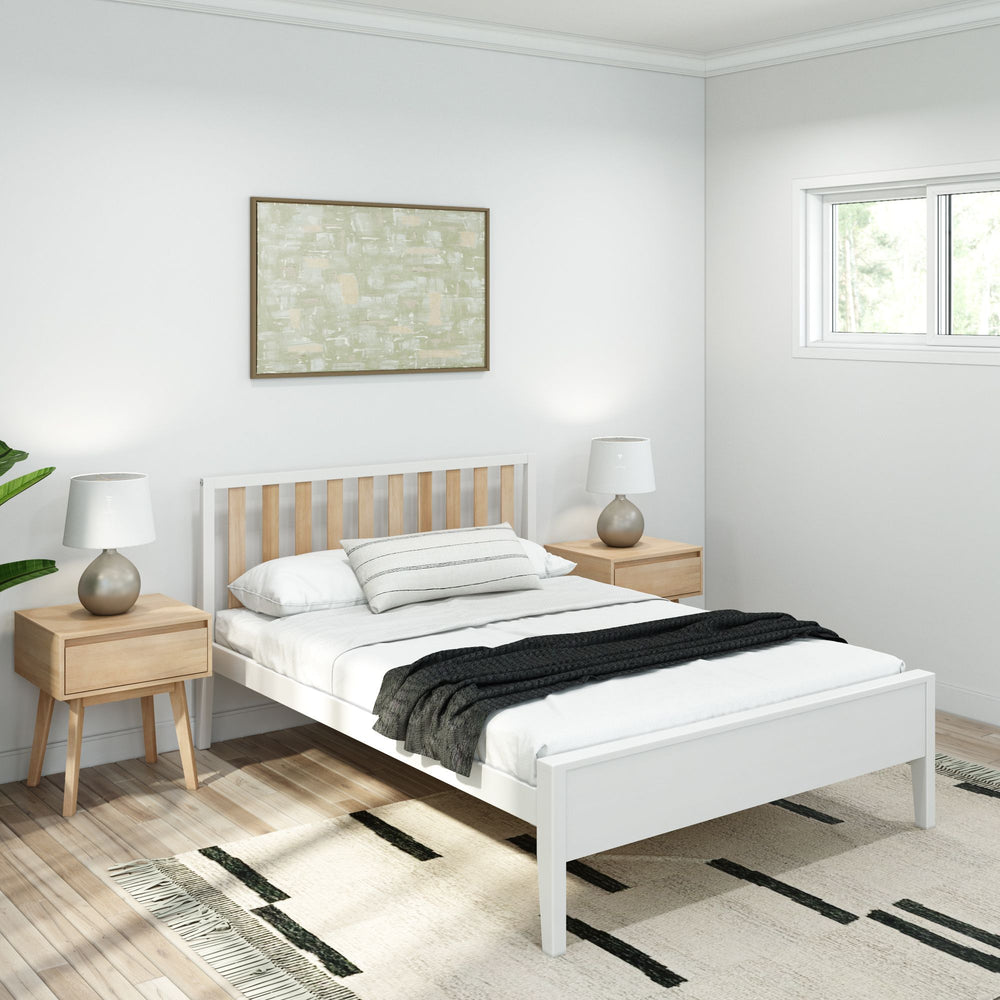This image captures a modern, minimalist bedroom bathed in natural light. The room features wooden flooring topped with a gray and white diamond-patterned rug. The centerpiece is a double bed with a white wooden frame and a low headboard accentuated with brown wooden slats. The bed is neatly made with white sheets, a white blanket, and a combination of large and narrow white pillows.

On either side of the bed, there are matching white wood nightstands with light-colored drawers. Both nightstands are adorned with white vases filled with flowers, ceramic items, and additional decor. One side table also holds a couple of books. Above the bed stands a row of narrow windows that allow sunlight to stream in, highlighting the serene ambiance.

Hanging from the ceiling is a modern gold chandelier with an open bulb design, consisting of three parallel lines of lights. The white walls are complemented by modern art pieces hung above the nightstands, adding a touch of sophistication to the room. The overall design is clean and contemporary, creating a peaceful retreat.